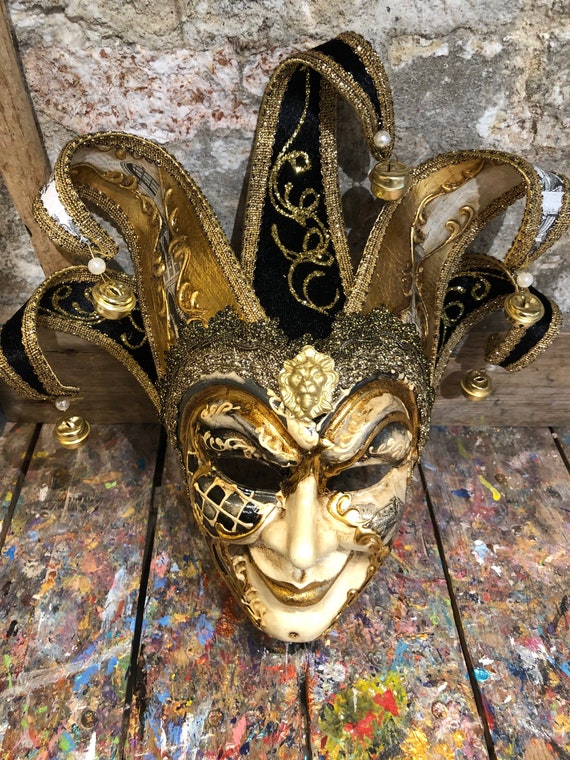The image showcases an elaborate, gilded mask reminiscent of a Joker on a deck of playing cards, but with a Mardi Gras flair. The mask features a striking combination of white, gold, and black, highlighted by intricate artwork and designs that include glittery swirls in silver and gold. The Joker's traditional hat has five fabric points, each adorned with golden bells and glittering accents, tapering downward. The mask's face is predominantly white with a sinister, upturned smile and slanted eyes, further accentuated by gold lips and a mask-like pattern around the eyes. A golden lion's face—with a detailed mane—adorns the center of the forehead, adding to the mask's opulent design. The mask rests on a weathered wooden deck splattered with multicolored paint drippings, characteristic of an artist's studio, and is set against an old brick wall.